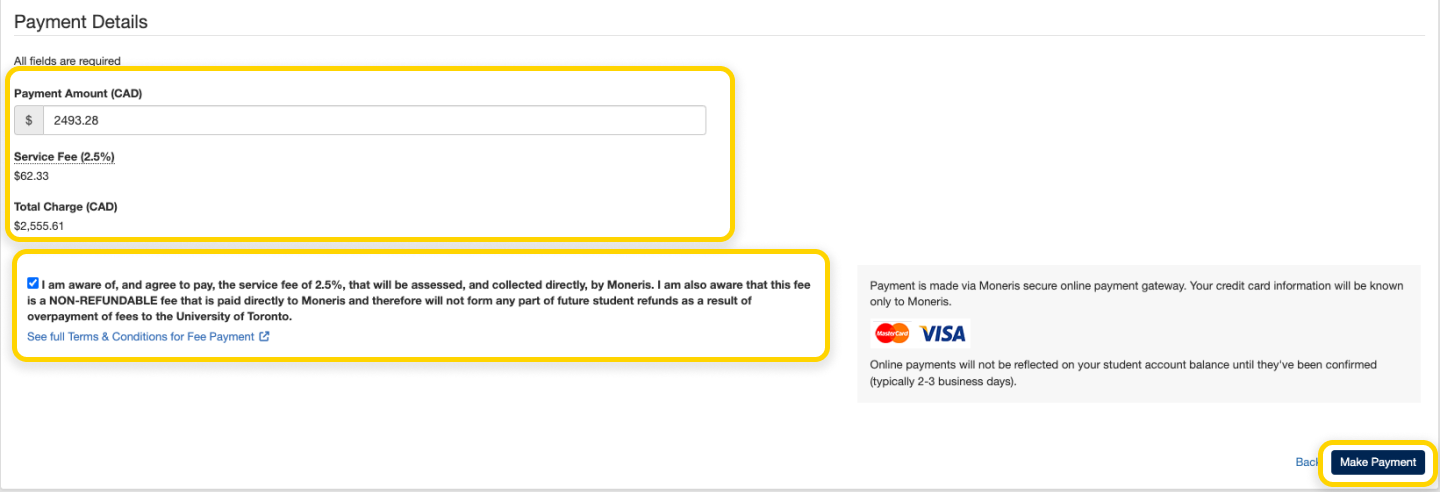A screen capture of a detailed payment detail page on a website. The background is predominantly white, with the text in black. At the top left corner, a bolded black header reads "Payment Details," followed by a gray horizontal line beneath it.

Immediately below this, a yellow-outlined rectangle contains a notice in small black text: "All fields are required." The next section starts with the label "Payment Amount (CAD)," which is bolded in black, and below it, there is a text area filled with the amount "2493.28" in black text.

Subsequently, the "Service Fee" is bolded, accompanied by "(2.5%)" in parentheses. Below this label, the fee amount "62.33" is listed. The "Total Charges" are then detailed, with "Total Charges (CAD)" appearing in black text and the total amount "2555.61" listed beneath it.

Following the total charges, there is another gray horizontal line. Below this, another yellow-outlined rectangle houses a blue box with a white checkmark and the text: "I'm aware of and agree to pay the service fee of 2.5%." Further information about the agreement for the University of Toronto payments is also provided.

In the bottom left corner, hyperlinked blue text states, "See full terms and conditions for fee payment," with an adjacent blue square containing an upward right arrow. On the right-hand side, the bottom corner features a rectangular gray area with the message: "Payment is made by a Moneris Secure Online Payment Gateway. Your credit card information will be known only to Moneris." This area also displays the MasterCard and Visa symbols. Below this, a notice indicates: "Online payments will not be reflected on your student account balance until they have been confirmed, typically two to three business days."

Finally, in the bottom right corner, there is a blue "Back" button, and next to it, a yellow-outlined black button with white lettering that says, "Make Payment."